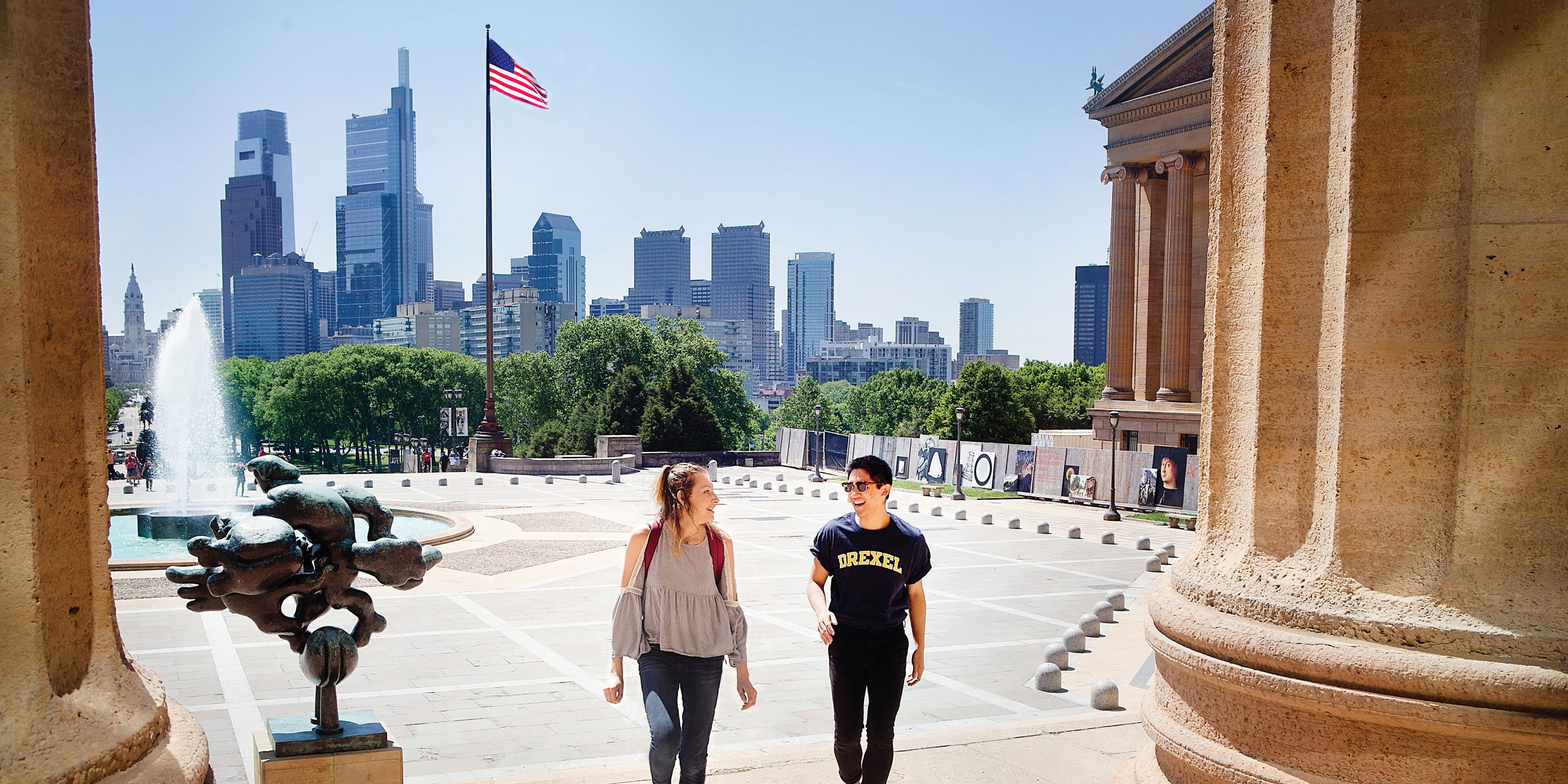This color photograph captures a vibrant scene at a college campus, with blue skies and a cityscape in the background, including tall gray buildings and a skyscraper skyline. An American flag waves atop a tall flagpole, anchoring the image’s patriotic elements. Dominating the image are two grand tan columns that evoke the grandeur of a governmental building, possibly reminiscent of a capital building. 

In the foreground, a male and a female student are walking up a sizable stairway. The male, with black hair, dons a t-shirt emblazoned with "Drexel," likely representing Drexel University, while the female, outfitted in jeans and a shoulder-less, long-sleeved shirt, carries a red backpack and looks at him with a smile, indicating they are engaged in a light-hearted conversation. To the left, water spews high from a circular fountain, adding a dynamic touch to the scenery. A statue base adorned with an eagle rises from the left foreground, contributing to the thematic grandeur. A nearby fence decorated with artwork and green trees further accentuates the lively, sophisticated campus atmosphere.